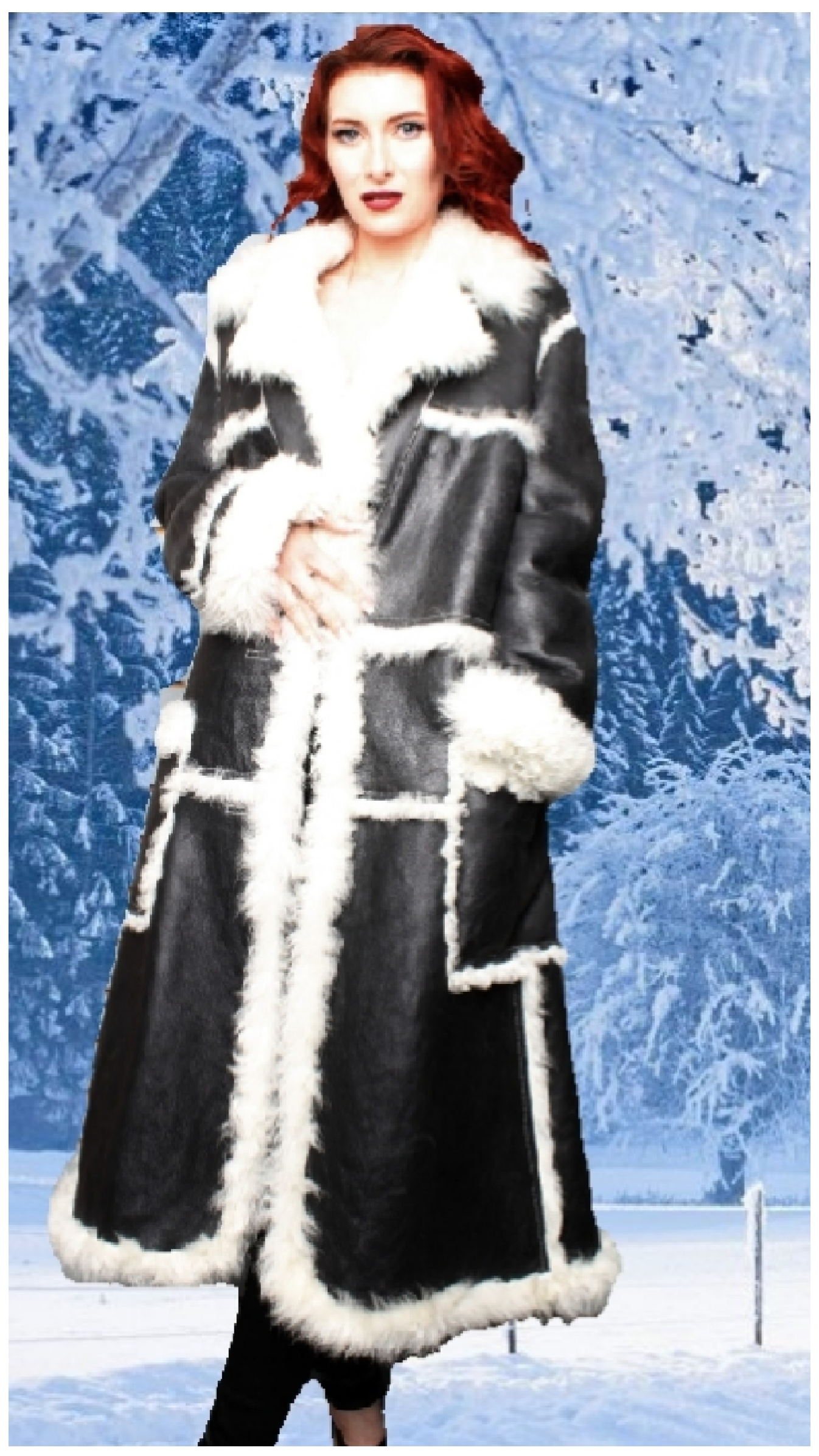This is an image of a woman with deep auburn red, curled hair and fair skin, giving the appearance of a model. She has dark red lipstick and is looking straight at the camera. She is wearing a light black or dark gray leather trench coat or sheepskin coat, exquisitely trimmed with white, furry, and feathery accents around the collar, cuffs, down the front, and along the bottom edges. The coat features distinctive angular square cut-outs also lined with the furry trim. The woman has her right hand resting above her abdomen, below her chest, while her left hand is tucked into a pocket, and her legs are crossed at the knee. The backdrop is a medium dark blue with white accents, depicting a frozen, wintery landscape with snow-covered ground and frost-covered branches. Although the background appears to be poorly Photoshopped, creating a somewhat artificial appearance, the overall ambiance suggests a chilly, snow-laden environment.